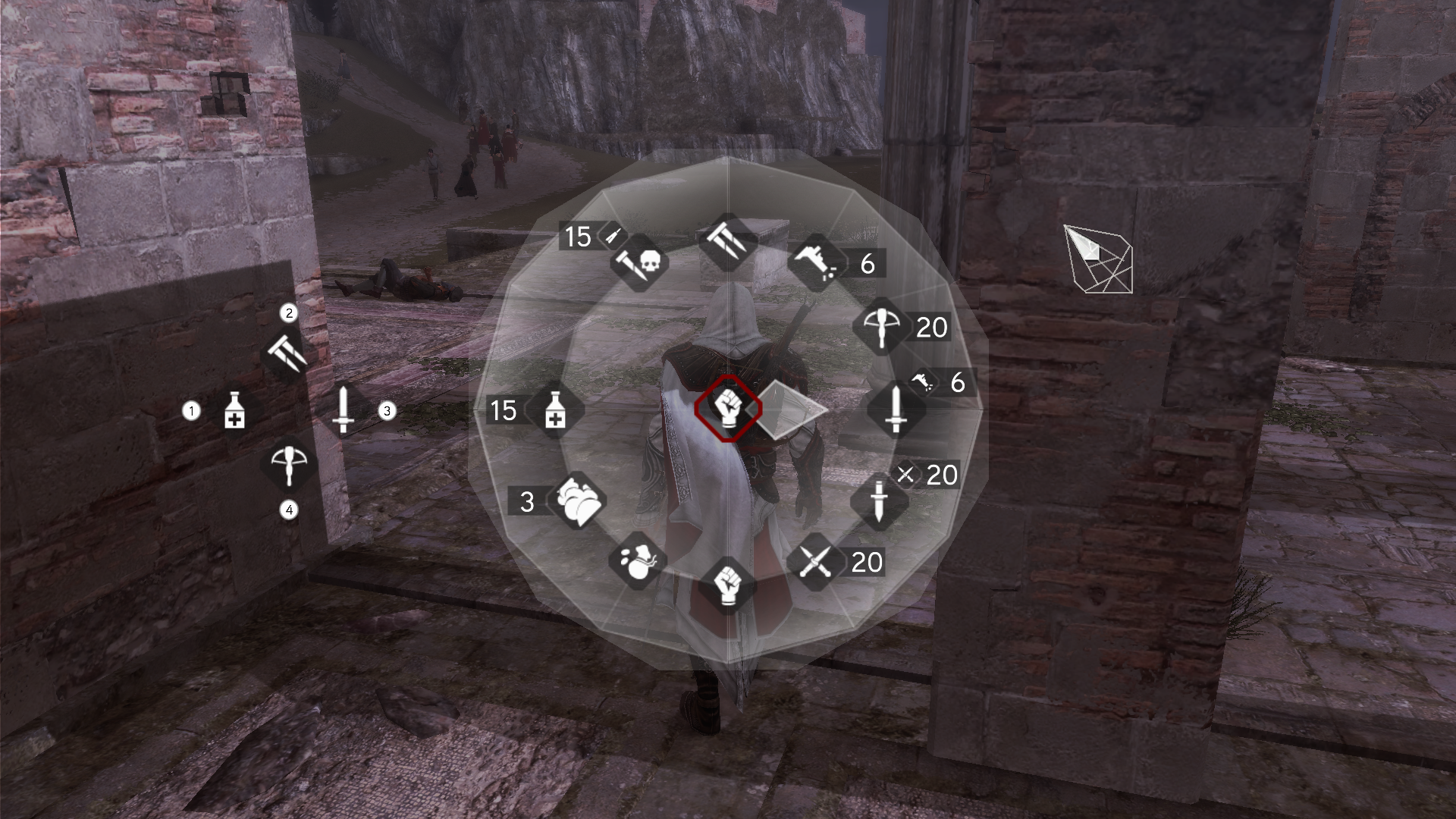In this screenshot from a video game, the central focus is on a cloaked figure, presumably the protagonist or main character. The figure, adorned in a white hooded cloak with red accents and gray armor over the shoulders, stands in what appears to be a brick and stone building. The environment is defined by its rugged brick and stone walls on the left, with an additional small pillar visible on the right, suggesting an ancient or medieval setting.

Above the character, a semi-transparent overlay screen displays the protagonist's skill set and inventory. This circular interface features various icons, each representing different abilities or items, surrounded by numerical values that likely indicate their quantity or level. On the left side of this overlay are four diamond-shaped icons: the top one depicts a bottle with a plus sign, possibly indicating a medicinal item, labeled with a "1"; to the right is a sword icon labeled with a "3"; at the bottom, a crossbow icon labeled with a "4"; and at the top, an icon resembling dual daggers.

Within the center of the circular overlay are additional icons: a sword, a crossbow, a shorter sword or dagger, two crossed knives, a fist, another medicine bottle, what appears to be a cloud, and a bag of money. Each icon is meticulously placed, providing the player with quick access to a variety of tools and abilities necessary for gameplay. The detailed interface and the character's intricate attire underline the game's focus on strategic resource management and immersive role-playing elements.